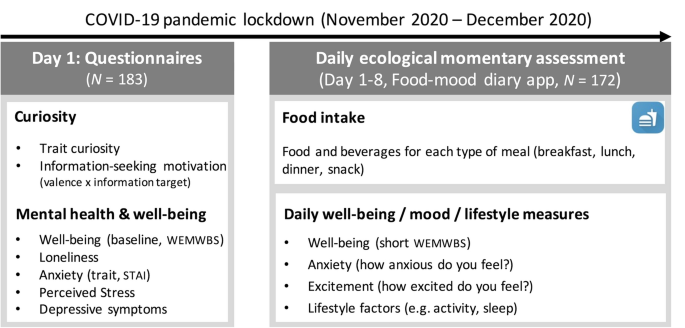The image depicts a detailed methodology diagram for a wellness survey conducted during the COVID-19 pandemic lockdown from November 2020 to December 2020. At the top, it notes the survey's timeframe. Below that, an arrow extends from left to right, highlighting two primary components of the study. 

On the left, a gray box titled "Day 1: Questionnaires (N=183)" summarizes the initial phase. This section includes two main categories: "Curiosity," covering aspects like Trait Curiosity and Information-Seeking Motivation (Valence X Information Target), and "Mental Health and Well-Being," with bullet points addressing Well-Being (Baseline WEMWBS), Loneliness, Anxiety (Trait STAI), Perceived Stress, and Depressive Symptoms.

On the right, the box titled "Daily Ecological Momentary Assessment (Day 1-8, Food/Mood Diary App, N=172)" outlines the daily tracking phase. This section is divided into "Food Intake," detailing food and beverage consumption for each meal (Breakfast, Lunch, Dinner, Snack), and "Daily Well-Being/Mood/Lifestyle Measures," which include indicators such as Well-Being (Short WEMWBS), Anxiety (How Anxious Do You Feel), Excitement (How Excited Do You Feel), and Lifestyle Factors (e.g., Activity, Sleep).

The diagram provides a clear visual representation of the study's structure, highlighting both the initial questionnaire data and the ongoing daily assessments to track changes in participants' well-being, mood, and lifestyle during the lockdown period.